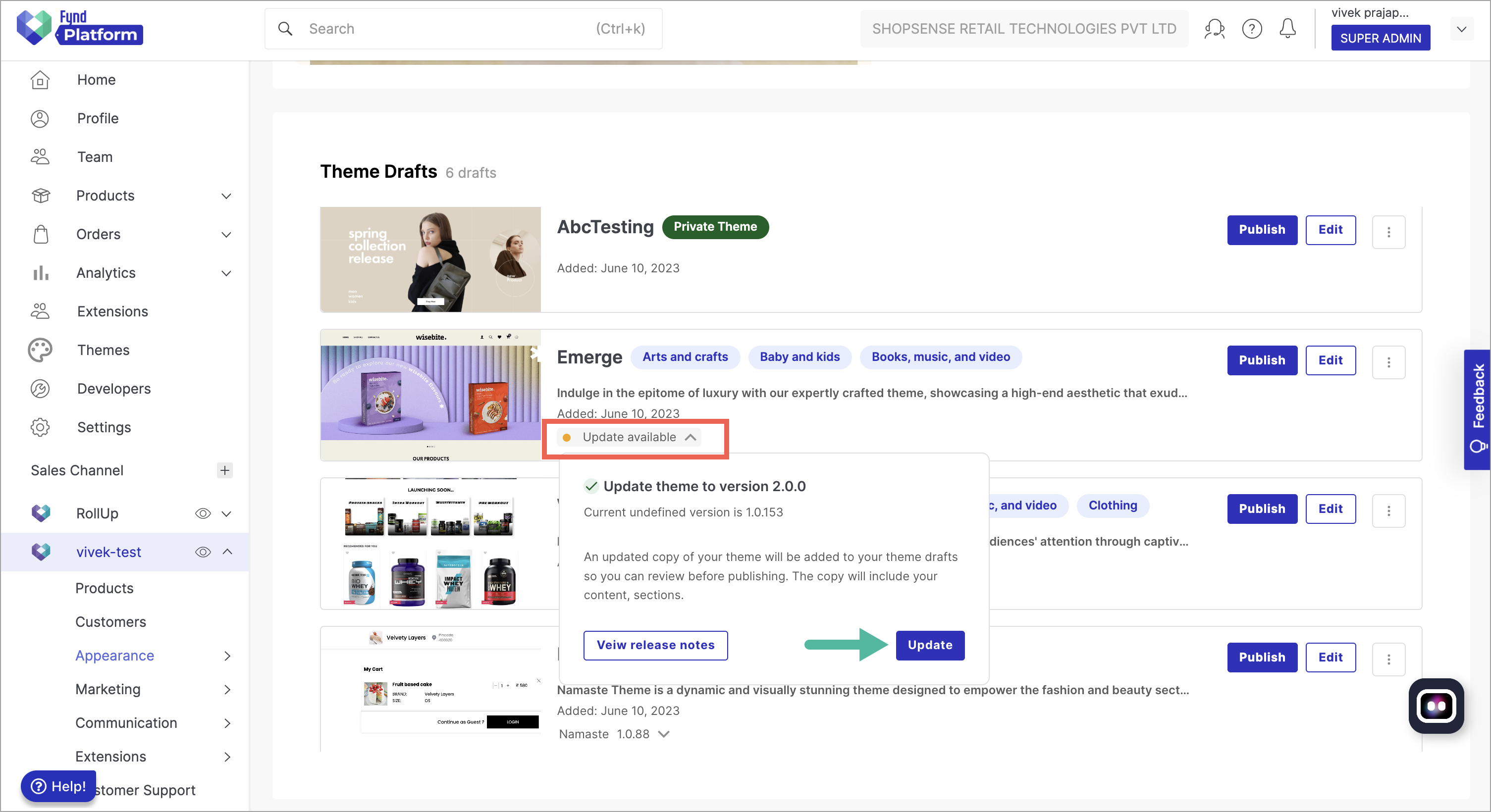**Screenshot of Fun Platform Web Page Interface**

The image depicts a detailed screenshot of a web page belonging to the "Fun Platform." The left-hand side features a vertical navigation column with a prominent blue rectangle in the top left-hand corner, labeled "Fun Platform." Within this rectangle is an icon of a heart composed of blue and green colors.

The sidebar contains a comprehensive menu with the following options:
- Home
- Profile
- Team
- Products
- Orders
- Analytics
- Extensions
- Themes
- Developers
- Settings
- Sales Channel

Further down, it includes additional sections:
- Viva
- Test
- Products
- Customers
- Appearance
- Marketing
- Communications
- Extensions
- Customer Support

At the very bottom of this sidebar, there's a blue button labeled "Help."

On the right-hand side, at the page's top, there's a search bar. Next to it is a brief text line that reads "ShopSense Retail Technologies PVT LTD." To its right, there is a user identification section displaying "Vivek P-R-A-P-A-J..." with the role "Super Admin" in blue text.

Beneath this top section, the main content area shows a white box titled "Theme Drafts," listing six drafts. The latest draft, "ABC Testing," is marked as a "Private Theme" with options to "Publish" and "Edit." Below it, there are theme categories listed: 
- Emerge
- Arts and Crafts
- Baby and Kids
- Books, Music, and Video

An enticing description follows: "Indulge in the epitome of luxury with our expertly crafted theme, showcasing a high-end aesthetic."

Suddenly, a pop-up notification appears within this area, prompting an update: "Update Theme to Version 2.0.0," with the current version noted as "undefined version is 1.0.153."